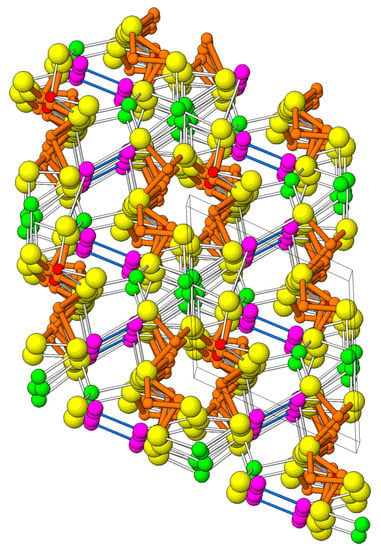The image depicts a vibrant and complex molecular structure set against a plain white background. The overall shape is a slightly tilted rectangular diamond, approximately four inches high and three inches wide. The molecules feature a rich array of colored spheres and rods that create a visually striking ensemble. Yellow, lime green, and magenta pink circles are prominently displayed, stacked atop one another to enhance the image's vibrancy. These colorful spheres are interconnected by rods of varying colors—mostly in light gray and navy blue, but also in orange and blue.

Starting in the lower right-hand corner of the structure, small green spheres with white rods extend to large yellow spheres. The yellow spheres are further connected to small pink ones by blue rods. Thicker orange rods emanate from the top of the yellow spheres, leading to thicker spheres also in yellow. Throughout the image, smaller colored spheres—including yellow, pink, and green—connect to one another seemingly at random, contributing to the image's intricate and vibrant appearance. Overall, this arrangement of multicolored atoms and bonds forms a detailed and dynamic molecular representation.